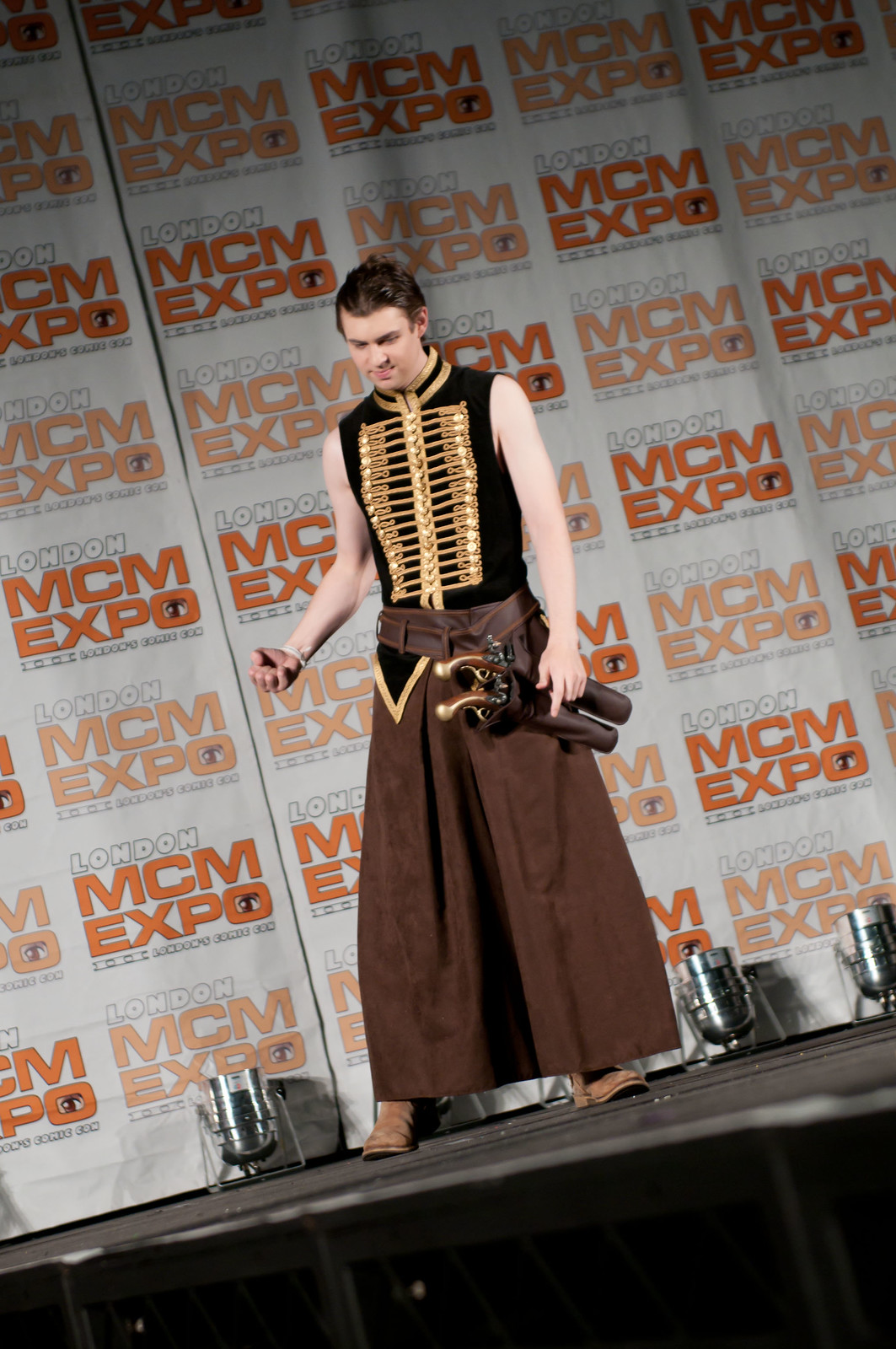A young Caucasian male, dressed as a fictional warrior, is posing on a black stage at the London MCM Expo, a Comic Con event. The backdrop behind him showcases a white banner with "London MCM Expo" in white and orange lettering. He wears a dark chocolate brown long skirt that reaches his feet, paired with light brown boots. His outfit includes a sleeveless, fitted black vest adorned with gold braided buttons and a tight collar. He sports a leather belt equipped with two old-fashioned musket pistols featuring golden-tipped handles and brown wooden stocks. The man has brown hair, a clenched right fist, and is looking down, capturing the essence of his character while stage lights illuminate the scene.